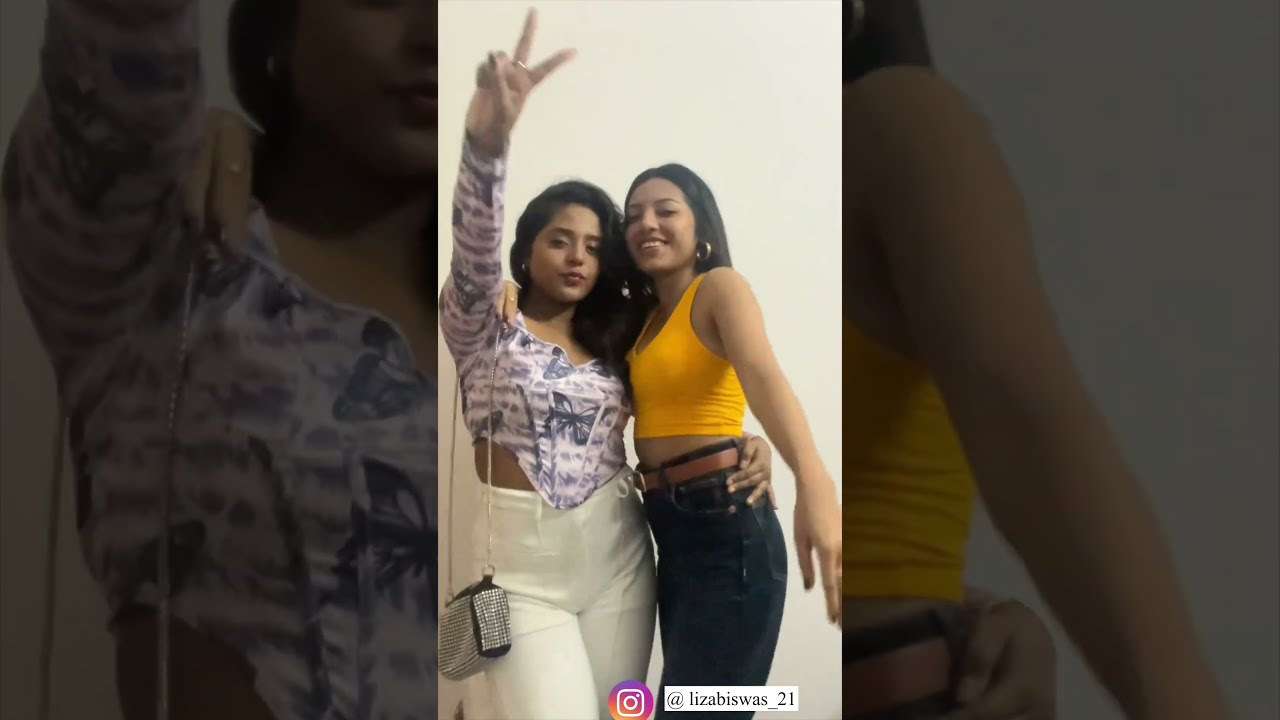In this photograph, two young women, possibly in their early 20s and of Spanish or Mexican descent, are posing together against a white wall. The woman on the left is dressed in white pants and a purple top adorned with purple butterflies. She is making a peace sign with her left hand, which has a ring on the middle finger, and has a sparkly, studded shoulder bag slung over her right shoulder. Her long black hair cascades down her back, and her left arm is affectionately around the waist of her friend. The woman on the right is wearing blue jeans and a yellow tank top that reveals her midriff, accented by a brown leather belt. She also has long black hair and is sporting hoop earrings. Both women are smiling warmly at the camera, enjoying the moment together as friends. The image is slightly blurry, especially around the white wall in the background, which has an Instagram link at the bottom.